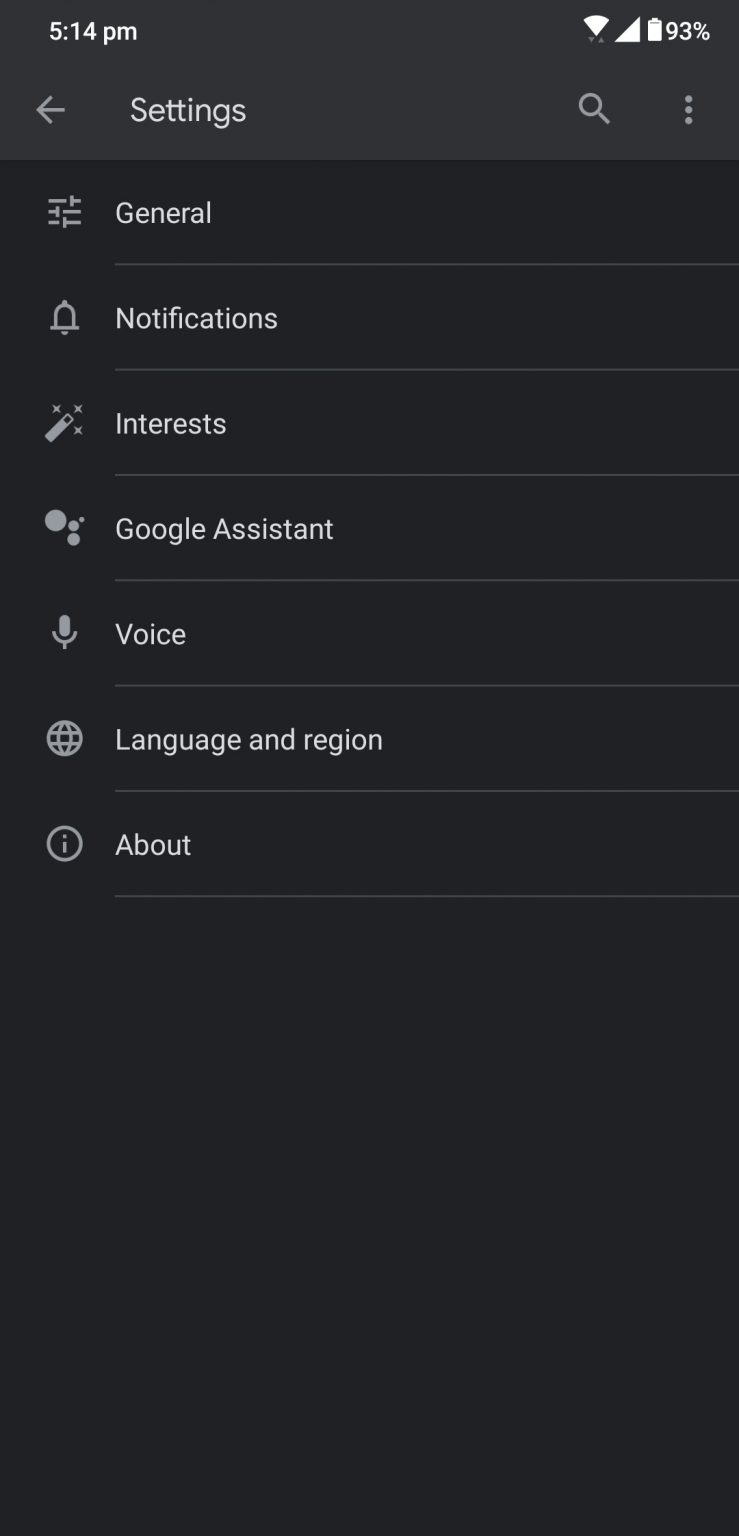The image is a screenshot taken from a cell phone, displaying the settings page. At the top left corner, the time is shown as 5:14 PM, while the top right corner indicates the battery level at 93%. The settings are organized into several sections, each separated by a faint gray line.

1. **General**: Displayed at the top of the visible list with no icon beside it.
2. **Notifications**: Represented by a bell icon.
3. **Interests**: Accompanied by an icon resembling a magic wand.
4. **Google Assistant**: Indicated with an icon of various gray balls in different sizes.
5. **Voice**: Marked by a microphone icon.
6. **Language and Region**: Shown with a globe icon.
7. **About**: Featuring a lowercase "i" within a gray circle.

The bottom part of the image is black, obscuring any further details.